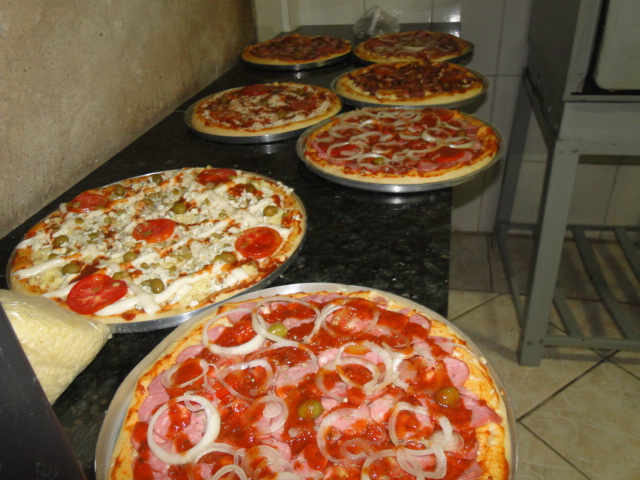This color photograph depicts a black and light gray marble table laden with seven completely whole, freshly baked pizzas still in their silver pans. Each pizza showcases a variety of toppings: one is adorned with Canadian bacon and large white onion rings, another features pepperoni and sausage, and yet another is covered with an assortment of vegetables including tomatoes, cheese, and olives. A bag of cheese, possibly Parmesan, rests near the bottom left corner of the table. The setting appears to be indicative of a restaurant or catering function, as suggested by the pristine, recently-out-of-the-oven appearance of the pizzas.

The surrounding environment includes a tan and brown tiled floor complemented by similarly colored tile walls. A gray shelving unit or possibly part of a pizza oven is partially visible on the right side of the image. The background also includes a white and brown hued wall on the left. In addition to the pizzas, a clear bag is seen at the far end of the table, though its contents remain indistinguishable from this distance. The scene reflects a carefully prepared presentation, emphasizing the variety and abundance of pizzas available.